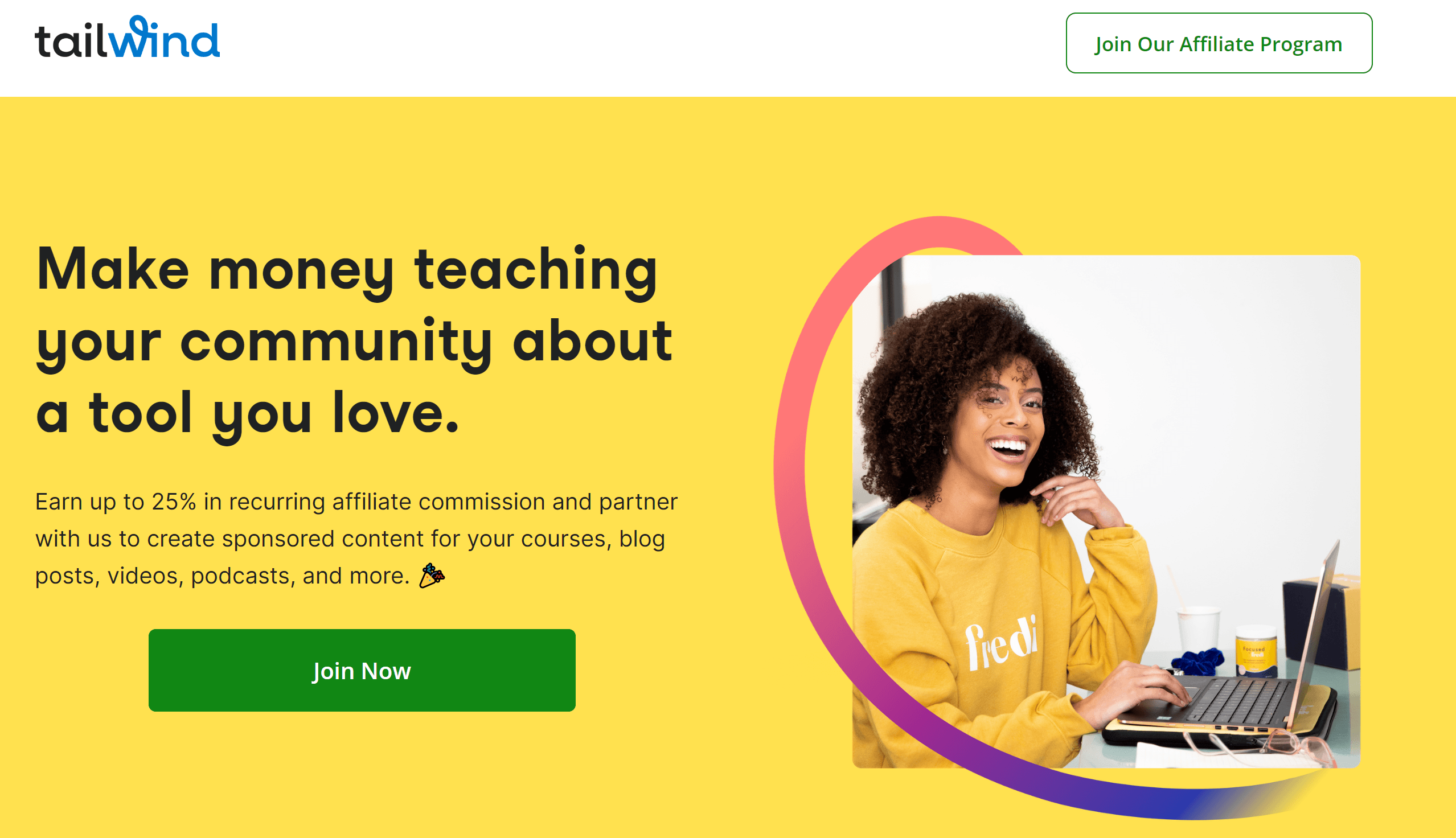Screenshot of a website with a layout optimized for desktop or laptop screens, characterized by long rectangular sections. The majority of the page features a bright yellow background. At the top of the image is a white banner, displaying the company's name, Tailwind, with "TAIL" written in black lowercase letters and "WIND" in blue cursive text. To the right on the banner, there is a prominent "Join Our Affiliate Program" button.

Dominating the yellow section, a square picture of a young Black woman is positioned on the right side. She sports a big curly hairstyle and a bright, genuine smile while wearing a yellow sweater that matches the background. In front of her is an open laptop, also yellow. She appears to be engaging directly with the viewer.

On the left side of the image, there is a prominently displayed text that reads: "Make money teaching your community about a tool you love. Earn up to 25% in recurring affiliate commission and partner with us to create sponsored content for your courses, blog, videos, podcasts, and more." Below this message is a green "Join Now" button, suggesting an opportunity to become involved in an affiliate program, potentially for creating and sharing content.